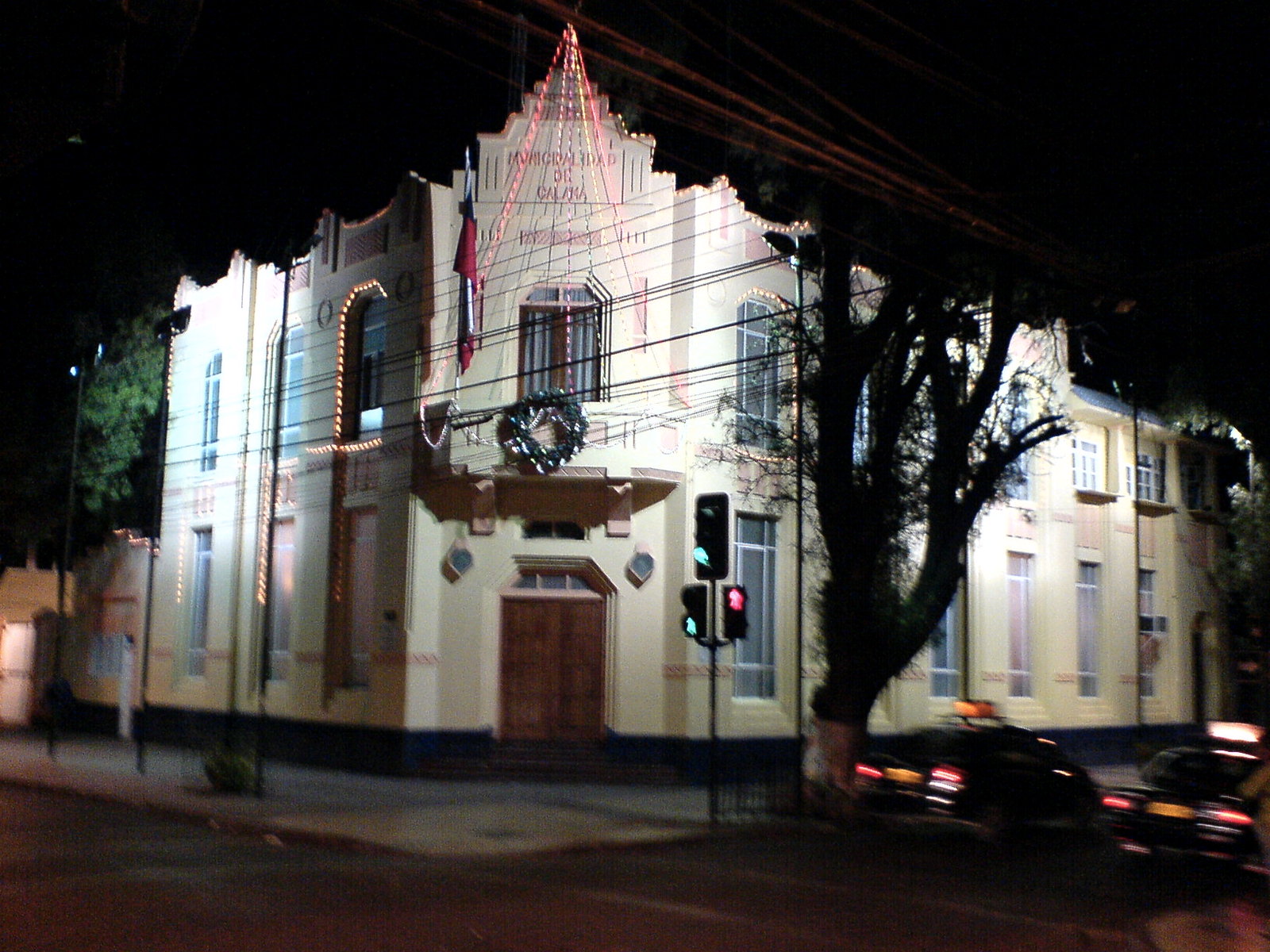This nighttime photo captures the exterior of a building taken from a diagonal angle across the street. The sky is pitch black, highlighting the festive ambiance created by the Christmas decorations adorning the building. A large tree, cast mostly in shadow, stands in front of the structure. Blurry taxis pass by on the street, emphasizing the stillness of the building itself.

Central to the image, the building features long, arched windows along the first floor, each framed by three smaller panes on both the top and the bottom, with a larger central pane. Christmas lights, glowing in shades of yellow and red, outline these windows and extend up to the pointed peak of the building’s front. A balcony above the wooden double doors—set at a corner entrance—hosts a lit wreath with multicolored lights. Additionally, a Christmas tree design, made of lights, projects outward from the balcony, adding to the cheerful holiday display. The text on top of the building remains too blurry to decipher, adding a bit of mystery to this charming seasonal scene.